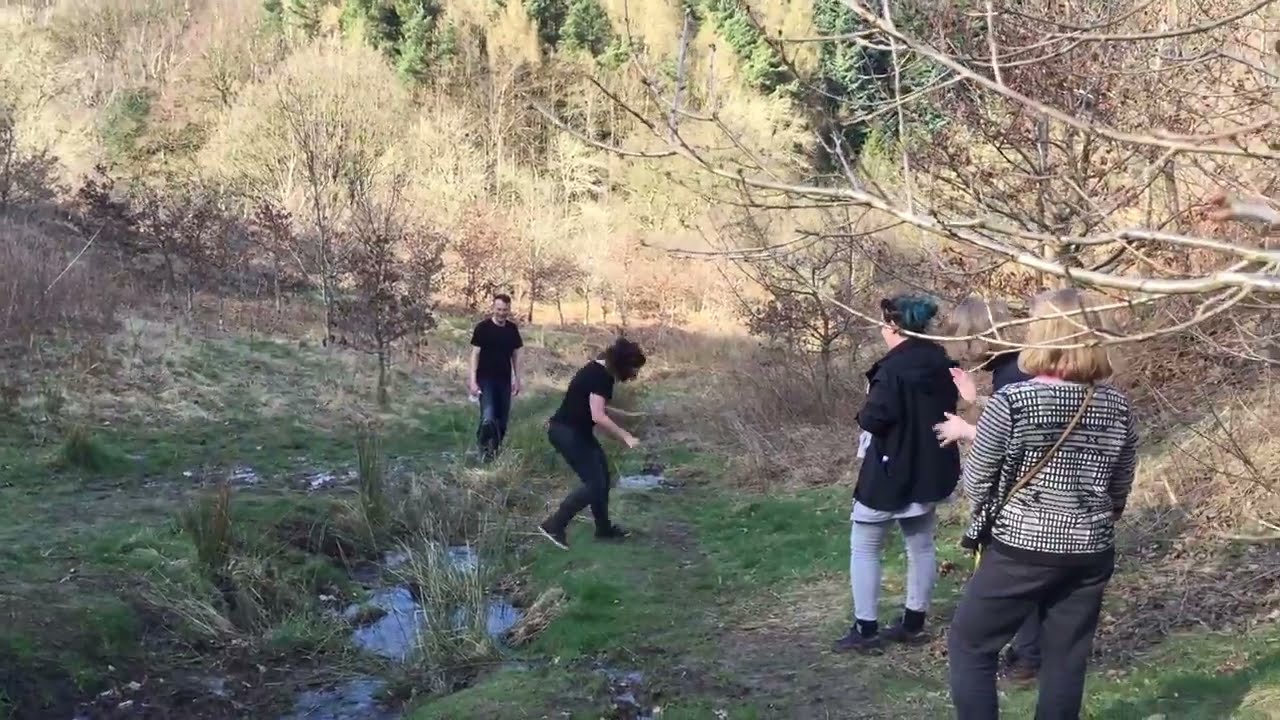A group of five friends is captured mid-hike in this outdoor scene, possibly during early spring, late fall, or late winter, suggested by the mix of green grassy terrain and bare trees in the background. They are traversing a grassy trail with noticeable elevation differences, as a narrow creek with a small waterway cuts across their path. One of the hikers, a young woman dressed in all black, is in the midst of hopping over the creek while another person, also clad in black, looks prepared to follow. Behind them stands a young man in a black t-shirt and blue jeans, watching their progress with either applauding enthusiasm or snapping a photo. Further back, another woman with blonde hair is also seen taking a picture. She wears a gray print jacket and black pants, complemented by a black and white handbag. In the center of the group is an older woman with her back to the camera, dressed in a black jacket and blue jeans. The hikers' outfits mainly consist of black and gray, blending with the subdued colors of the environment. The backdrop features a blend of coniferous green trees and the bare branches of deciduous trees, setting a serene and candid scene of friends enjoying a hike together.